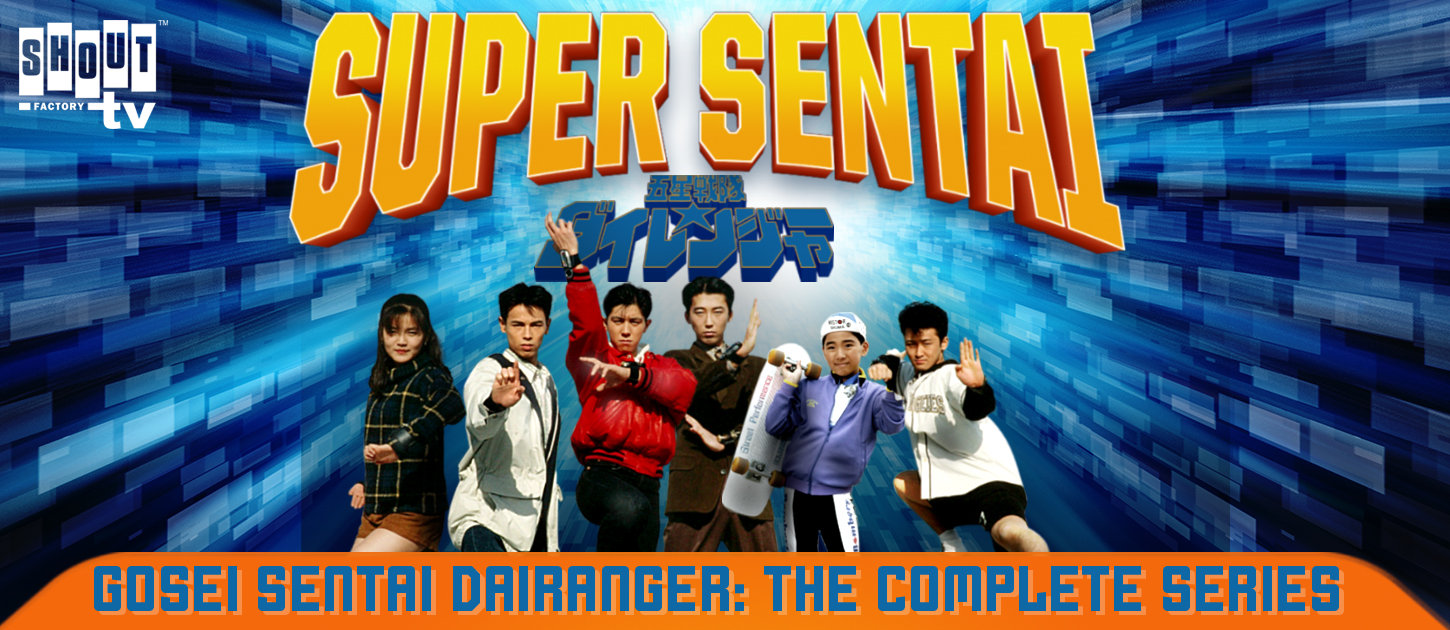The promotional image for the TV show features a dynamic composition with vivid colors and bold text. In the top left corner, multiple white letters within rectangles spell out S-H-O-U-T, followed by a line of white text reading "Factory TV." Dominating the center of the image, the title "Super Sentai" is displayed in large, curved orange font. Beneath it, two lines of blue Asian characters provide additional context. 

At the bottom center, six characters strike various martial arts poses against a fast-moving blue background. From left to right, the characters include: a woman in a black shirt and brown shorts, a man in a white Kung Fu outfit, a boy in a white jacket and black pants, a man in a brown outfit, a boy holding a skateboard in a light blue jacket and multicolored pants, and another boy who appears to be jumping in the air, dressed in a large white shirt and black shorts.

An orange banner at the bottom of the image features blue text that reads, "Gosei Sentai Dairanger The Complete Series." The vibrant promotional design effectively captures the energy and action of the TV show.